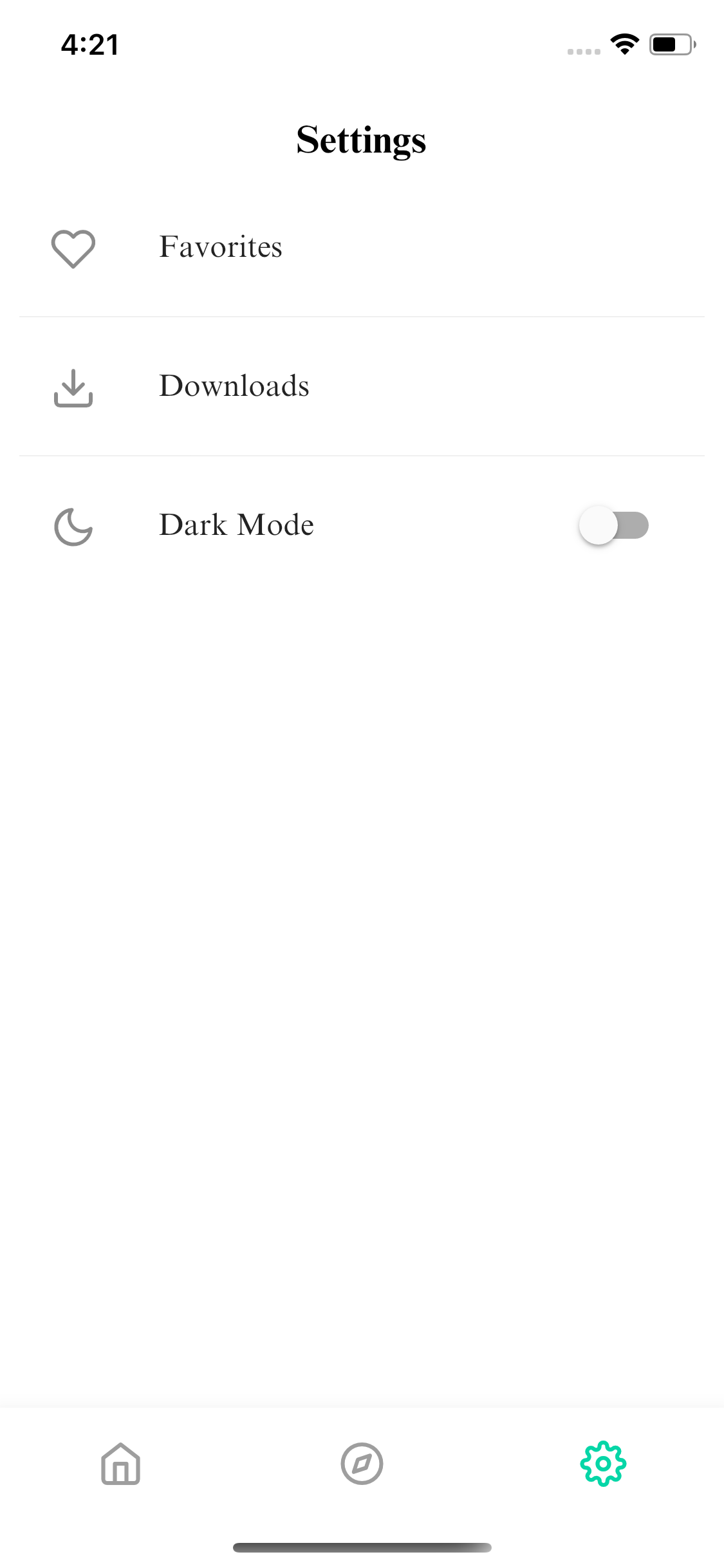A detailed screenshot reveals a user interface on a white background. In the top right corner, the time is displayed as 4:21. Adjacent to it are three horizontal gray dots representing a menu. The interface features several icons: a heart symbol indicating favorites, a download button, and a moon icon signifying dark mode. The dark mode toggle switch is currently set to off. Additionally, there is an image of a house and a compass, denoting home and navigation functionalities respectively. A conspicuous green settings icon is also present. At the bottom center of the screen is a horizontal gray bar.